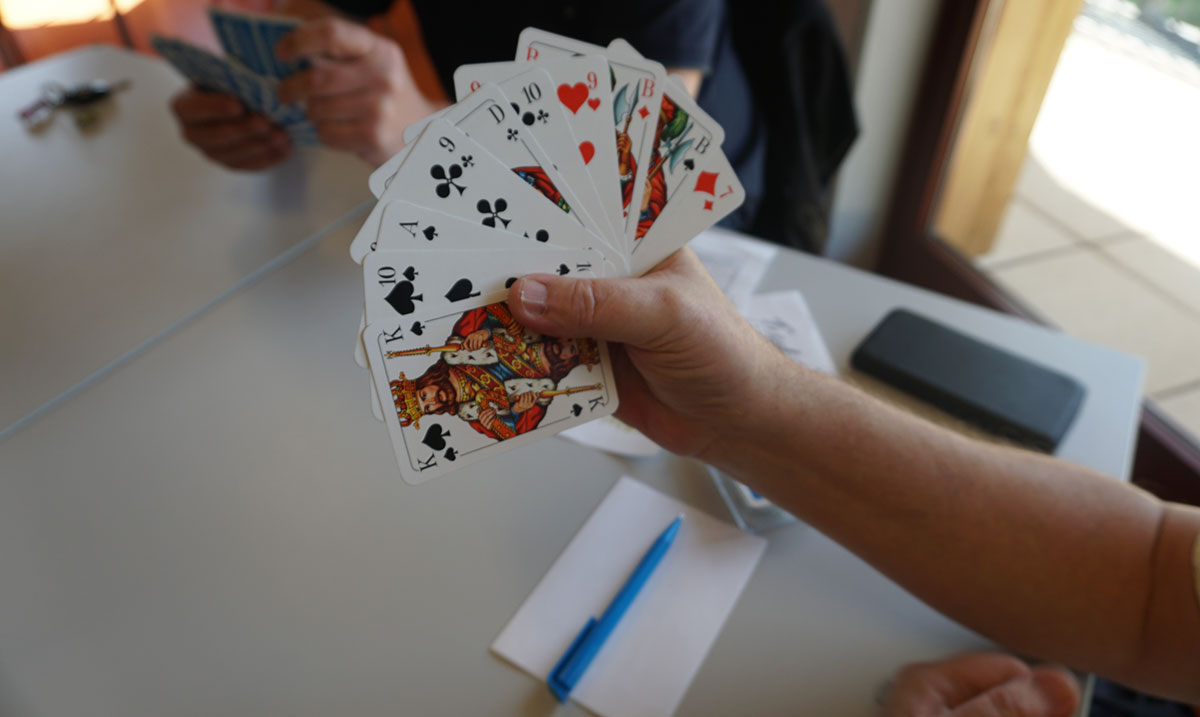The image captures a scene at a card game table, focusing on one player's hand. The setting appears to be indoors, adjacent to a patio with a glass door that extends to the floor, providing a clear view outside. The player's hand, identified by its masculine features and light arm hair visible from the hand down to the elbow, holds a set of playing cards. The cards are as follows: the King of Spades, the 10 of Spades, the Ace of Spades, the 9 of Clubs, an indistinct card, the Jack of Clubs, the 10 of Clubs, the 9 of Hearts, the 8 of Diamonds, another Spade marked with a "B," and the 7 of Diamonds. On the table lies a folded piece of paper and a blue ink pen, suggesting that they might be keeping score of the game.